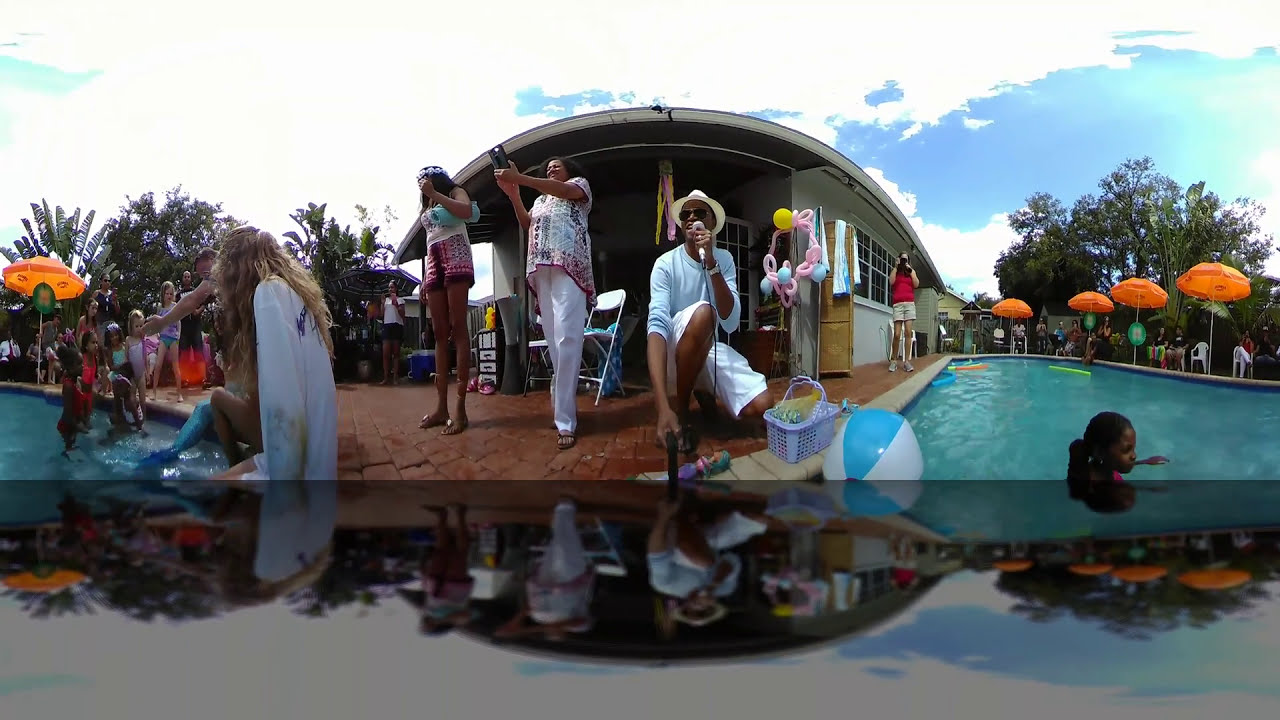The image captures a lively pool party at what appears to be a resort hotel. The pool is partially visible and not overly crowded, indicating that the party is spread out across different sections. People of all ages, shapes, and sizes are enjoying the sunny summer day, lounging by the pool and swimming. There's a festive atmosphere with a man holding a microphone, possibly acting as a DJ, engaging the crowd. He wears a white hat, pale blue shirt, and white shorts, and is holding a selfie stick.

In the center of the image, three people dressed in white pants and shirts, and one woman in red, are standing in front of a pool house, seemingly lost in thought as they look into the distance. The pool house acts as a backdrop, lending a central focal point to the scene. There are also colorful details: a young black girl with her hair in a ponytail is in the pool on the right side, accompanied by a blue and white beach ball and a purple basket. 

Bright orange umbrellas line the pool, contrasting with the deep green foliage of the surrounding bushes, while trees frame the scene. The sky above is a picturesque blue with scattered white clouds, enhancing the vibrant, carefree ambiance of the gathering. Some people are seen taking pictures, encapsulating moments of joy and the overall celebratory mood of the occasion.